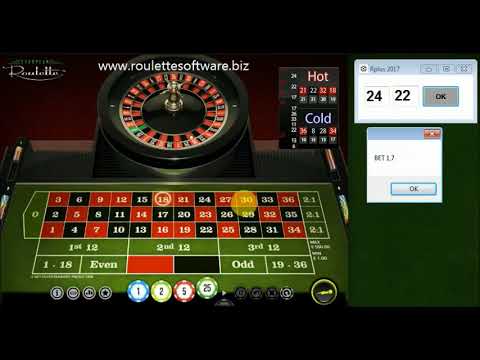The image is a detailed screenshot of an online gambling roulette game hosted on www.roulettesoftware.biz, visible in white font at the top of the image. The casino game interface is prominently displayed, with a green digital roulette table on the left side of the image featuring red and black numbered slots, as well as poker chips valued at 1, 2, 5, and 25. The roulette wheel itself is positioned above the board and is comprised of alternating red and black sections with a silver spinner in the center, adorned with a glow around the number 30 and a circle around 18. 

To the right of the roulette table, the screen is divided into two separate windows. The first window includes a scoreboard or calculator displaying the numbers 24, 22, and a button labeled "OK." Below this, another window simulates a Windows computer interface with a message indicating "bet 1.7." Additionally, there are labels for "hot" and "cold" numbers near the scoreboards, presumably tracking the frequency of recent winning numbers. The top and bottom of the image are framed by long black horizontal bars, adding to the graphical layout of the screen. The entire setup points to an interactive and dynamic gambling platform with detailed tracking and betting options.